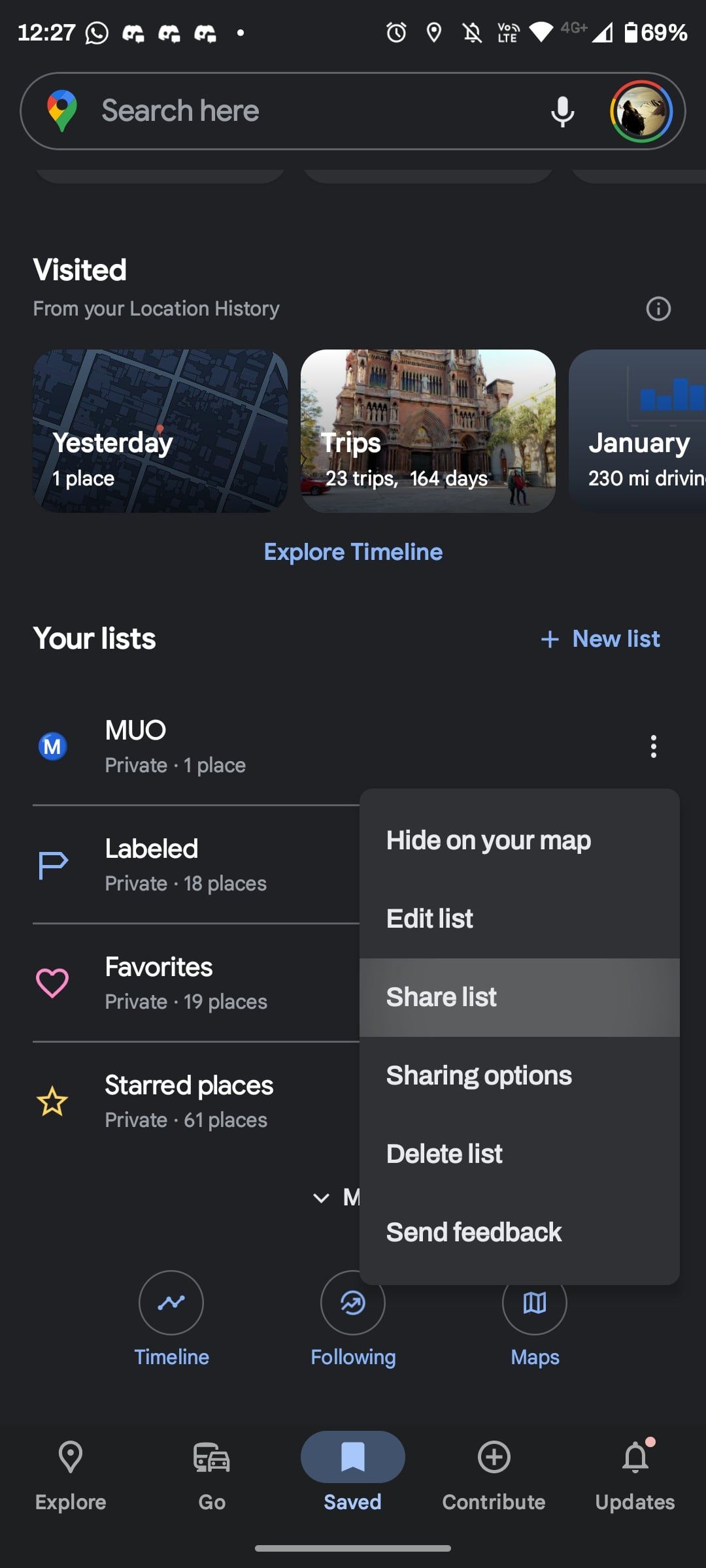A screenshot taken from a mobile phone displaying a Google app interface in night mode. The rectangular screen, typical of mobile phones, shows a black background with white text, indicating it's in night mode. At the very top, the status bar reveals the time as 12:27 along with various icons: a WhatsApp logo, an Android icon, an alarm clock, GPS, VoLTE, Wi-Fi indicating 4G connectivity, and a battery level at 69%.

The main content of the screenshot features a Google search bar at the top, with the user's profile partially visible. Below the profile, it mentions "location history" with details about recent activities: "Yesterday, 1 place," "23 trips, 164 days," and a snippet showing "January, 230 miles driving." Further down, the options "Explore Timeline," and various lists such as "Your lists," "M, U, O," "Favorite," "Starred places," "Highlighted starred places," and "Shared lists" are visible, providing an organized view of the user’s location data and personal lists.